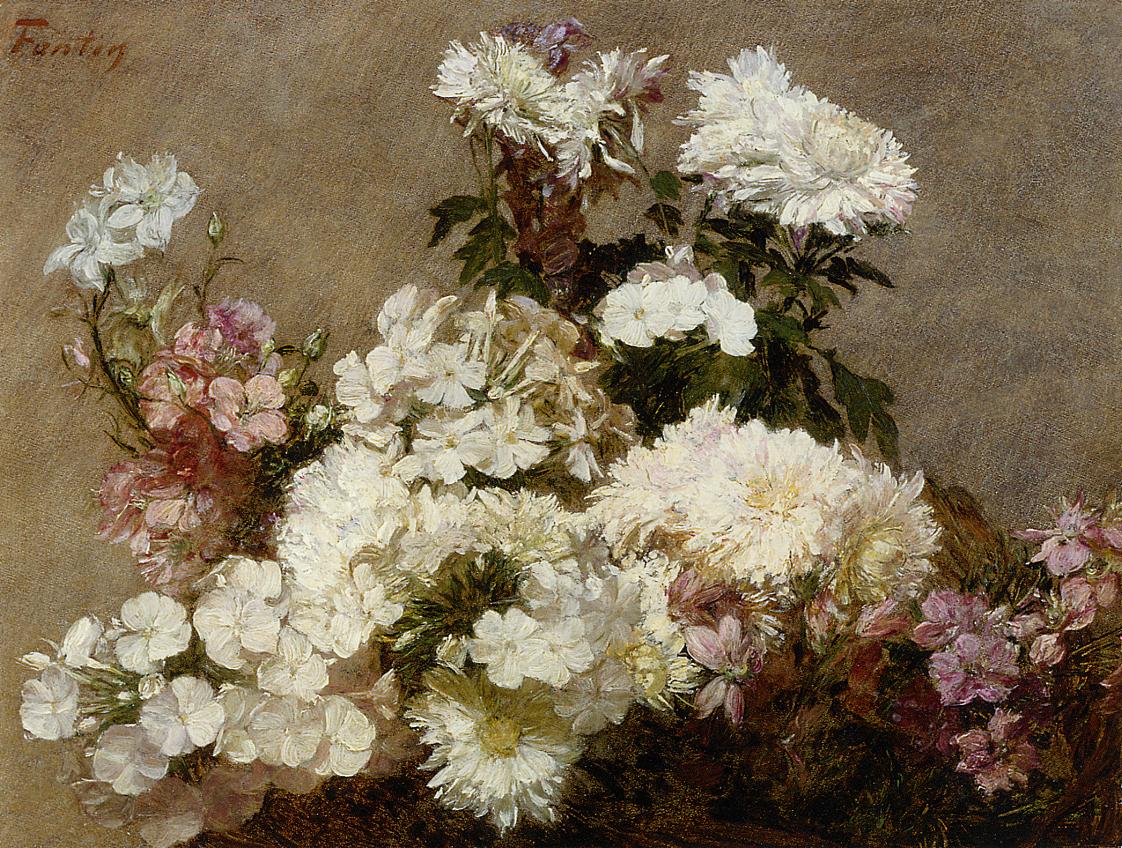This realistic oil painting depicts a visually captivating bouquet of flowers, strategically arranged in a triangular shape. The painting is set against a rough, grayish-brown background reminiscent of cement, which allows the vibrant flowers to be the focal point. Dominating the composition are large, white flowers, likely mums, that form the core of the bouquet. These are accompanied by smaller white flowers, resembling daisies, interspersed with subtle hints of green leaves and foliage that add to the natural feel of the arrangement.

To both the left and right sides of the bouquet, smaller, light pink flowers add a delicate touch of color and contrast against the predominantly white blooms. The flowers are densely packed, creating a layered effect with a band of large white flowers at the top tapering down into a mix of pink and purple flowers towards the bottom right corner. The overall appearance is both intricate and elegant, with each flower meticulously detailed to enhance their realism. Despite the rough background, the flowers' soft, delicate nature draws the viewer's eye, creating a striking still-life composition.